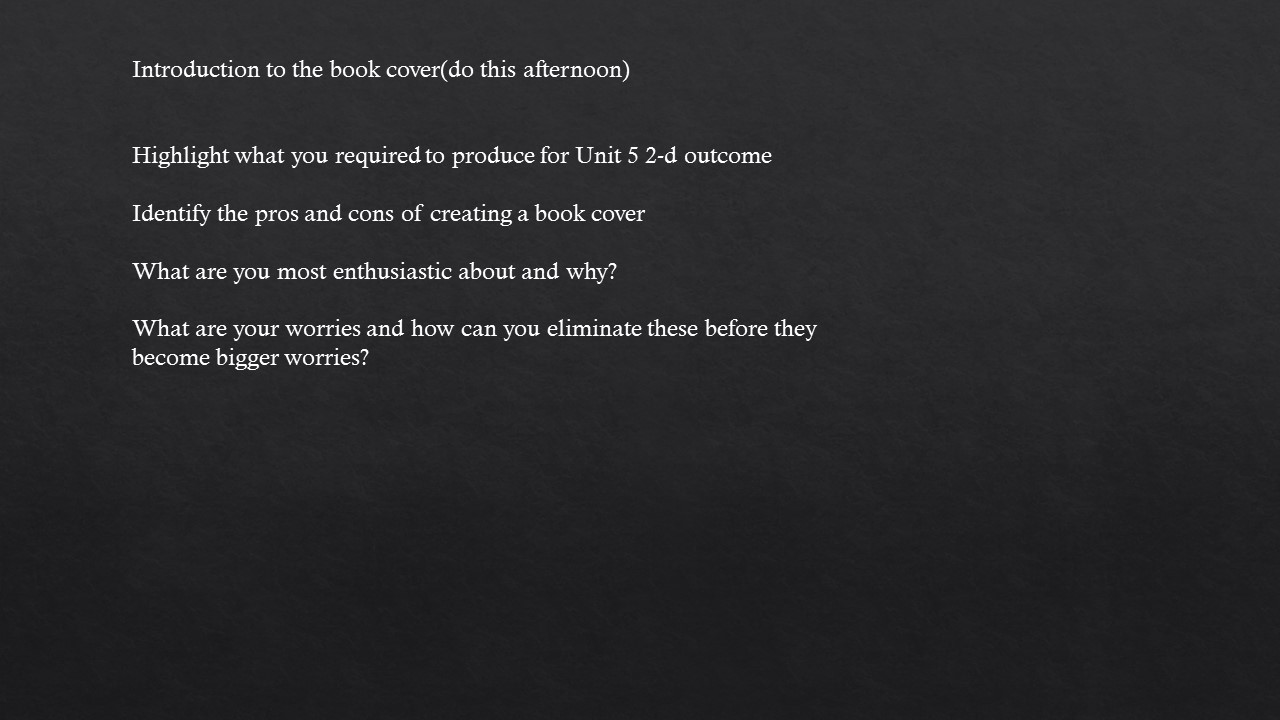The image displays a simple black rectangle, resembling a PowerPoint slide or classroom assignment. It features white text on a solid black background and measures around 3 by 5 inches, potentially extending up to 3 by 7 inches. The text, primarily located in the upper left corner, is formatted without periods at the end of each line, resembling an outline style. It reads: 

"Introduction to the book cover (due this afternoon). Highlight what you required to produce for unit 5, 2D outcome. Identify the pros and cons of creating a book cover. 

What are you most enthusiastic about and why? What are your worries, and how can you eliminate these before they become bigger worries?"

This concise list appears to outline the tasks and reflective questions for a book cover project, indicating its due date and the aspects students need to consider and address.